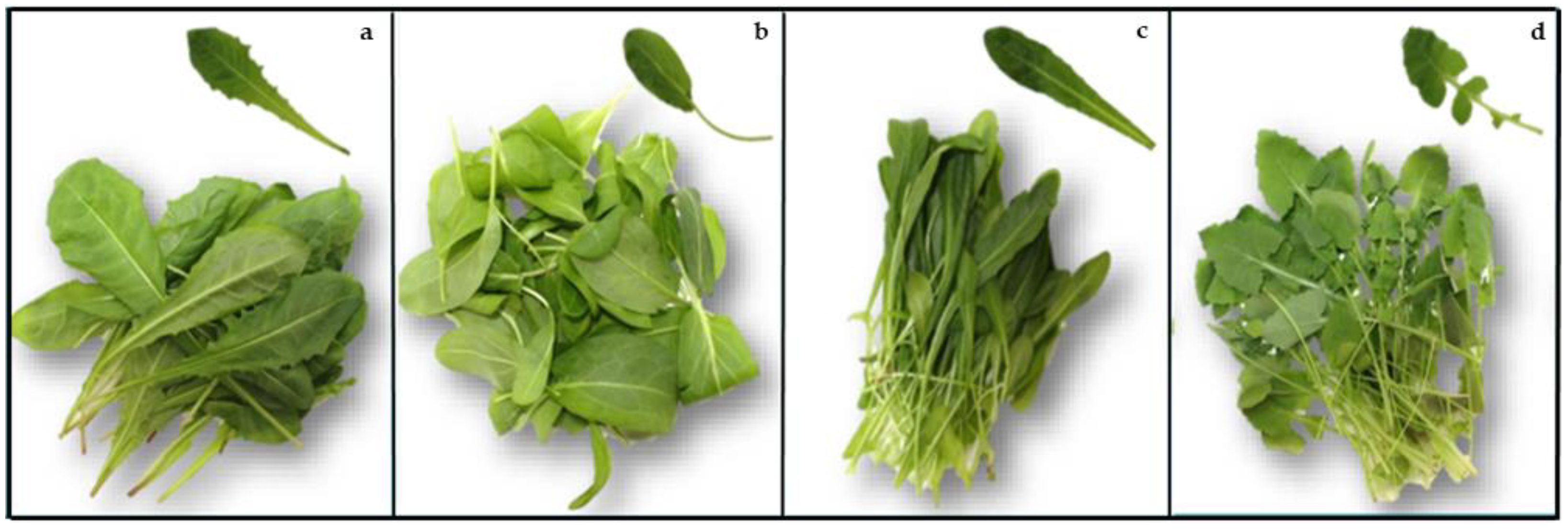This diagram is a horizontally oriented image composed of four labeled grids: A, B, C, and D, each displaying various types of lettuce leaves. The grids are arranged from left to right and are about two and a half times wider than they are tall. In each grid, a single representative leaf is placed towards the top, with a pile of similar leaves towards the bottom. 

Grid A features lettuce leaves that start thin and widen towards the edges, which are adorned with little pointy spikes. Grid B shows leaves with a cylindrical shape, smooth edges, and a long stem, displaying an oval form. Grid C contains smaller leaves that are also similar to those in A but are straighter, less curvy, and less spiky. Finally, Grid D has leaves that are segmented, resembling a clove or spade with multiple portions of the leaf blade. This progression from A to D illustrates increasingly smaller and more finely chopped leaves, demonstrating different stages of leaf preparation, likely for salad making.